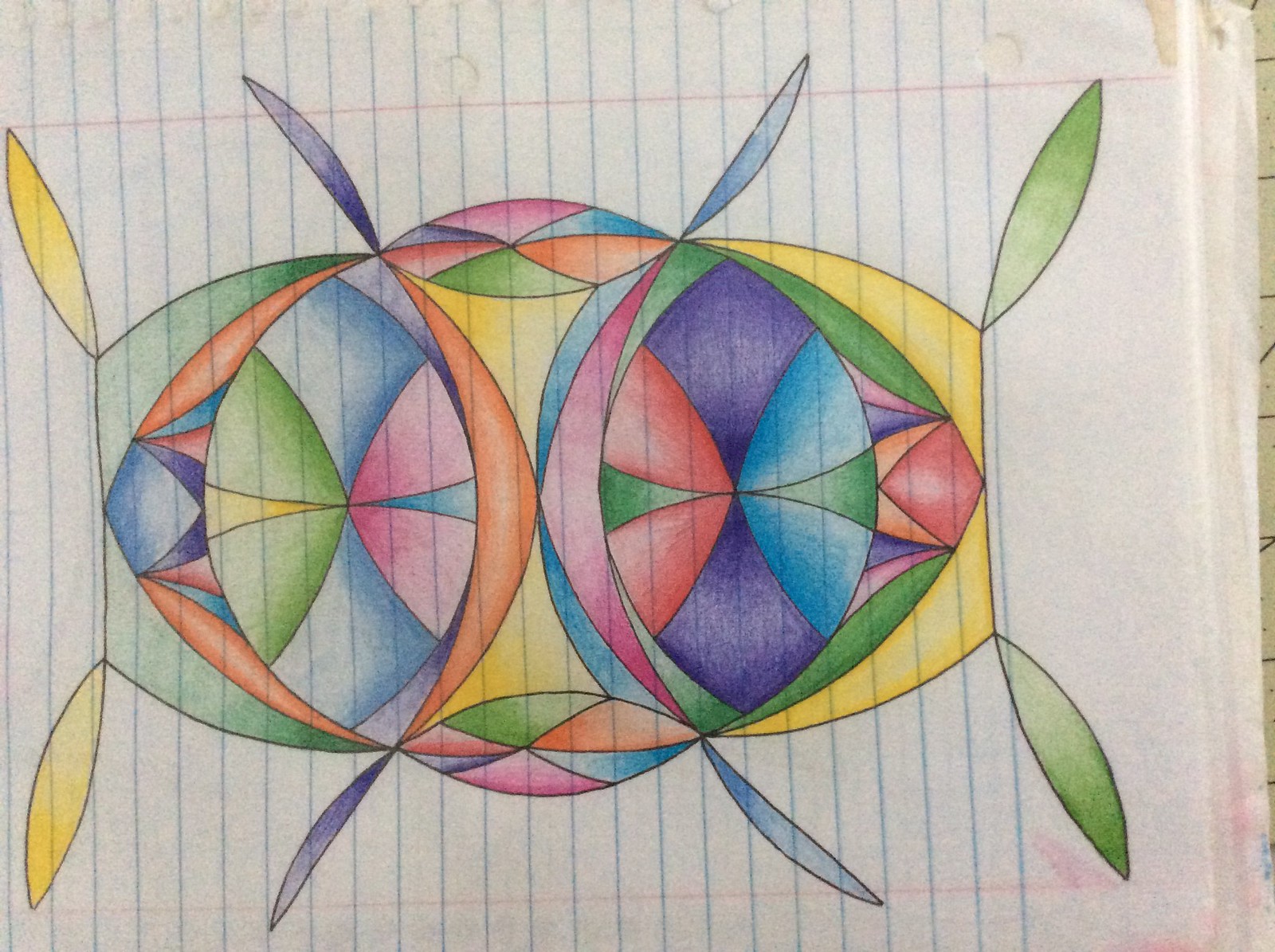A bird's eye view of a drawing on a ruled piece of paper, likely from a writing pad, is shown. The paper features a prominent white border at the top with vertically oriented ruled lines covering most of the page. The drawing is executed horizontally across these vertical lines, creating a striking geometric design. 

At each of the four corners of the drawing, there is a leaf-like petal emerging from a curved rectangular structure filled with interconnected circles. The curved rectangular structure, positioned toward the center from the corners, has convex top and bottom edges as well as outwardly curved sides that join seamlessly with small protruding circles. 

In the middle of the design, additional leaf-like petals are depicted, with four petals—two at the top and two at the bottom—colored blue. The overlapping circles within the geometric design are vividly colored in shades of blue, pink, green, yellow, orange, red, purple, and cyan, adding a lively and intricate detail to the abstract composition.